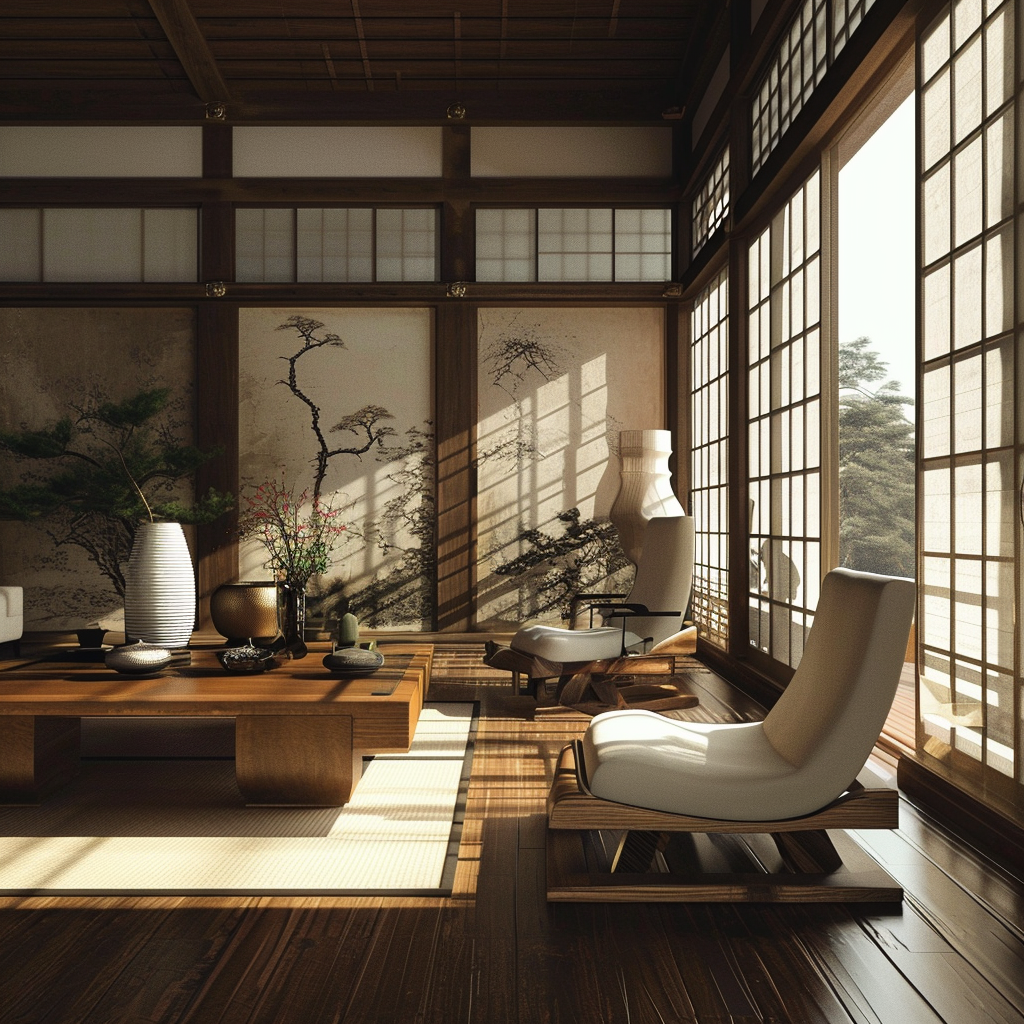This beautifully decorated, Japanese-style room exudes a serene and relaxing ambiance. It features high ceilings and dark wooden posts that contribute to an elegant, old-style Asian aesthetic. The wooden floors are made of smooth, dark planks, while sliding wooden doors with rice-paper-like panels allow daylight to illuminate the space. The walls are adorned with paintings of skinny trees and large plants, resembling Japanese artworks that cover entire panels of the wall, enhancing the room's charm.

The furnishings blend modernity with tradition. Two large, low-sitting lounge chairs with white cushions and wooden frames offer a cozy seating arrangement. A central, low wooden table adorned with big vases adds to the room’s sophisticated decor. The striking contrast between the modern furniture and the traditional elements of the interior creates a unique, harmonious atmosphere. The room opens to an area with trees, and the visible sky and natural daylight filtering through the doors add a touch of tranquility, making it a perfect sanctuary.